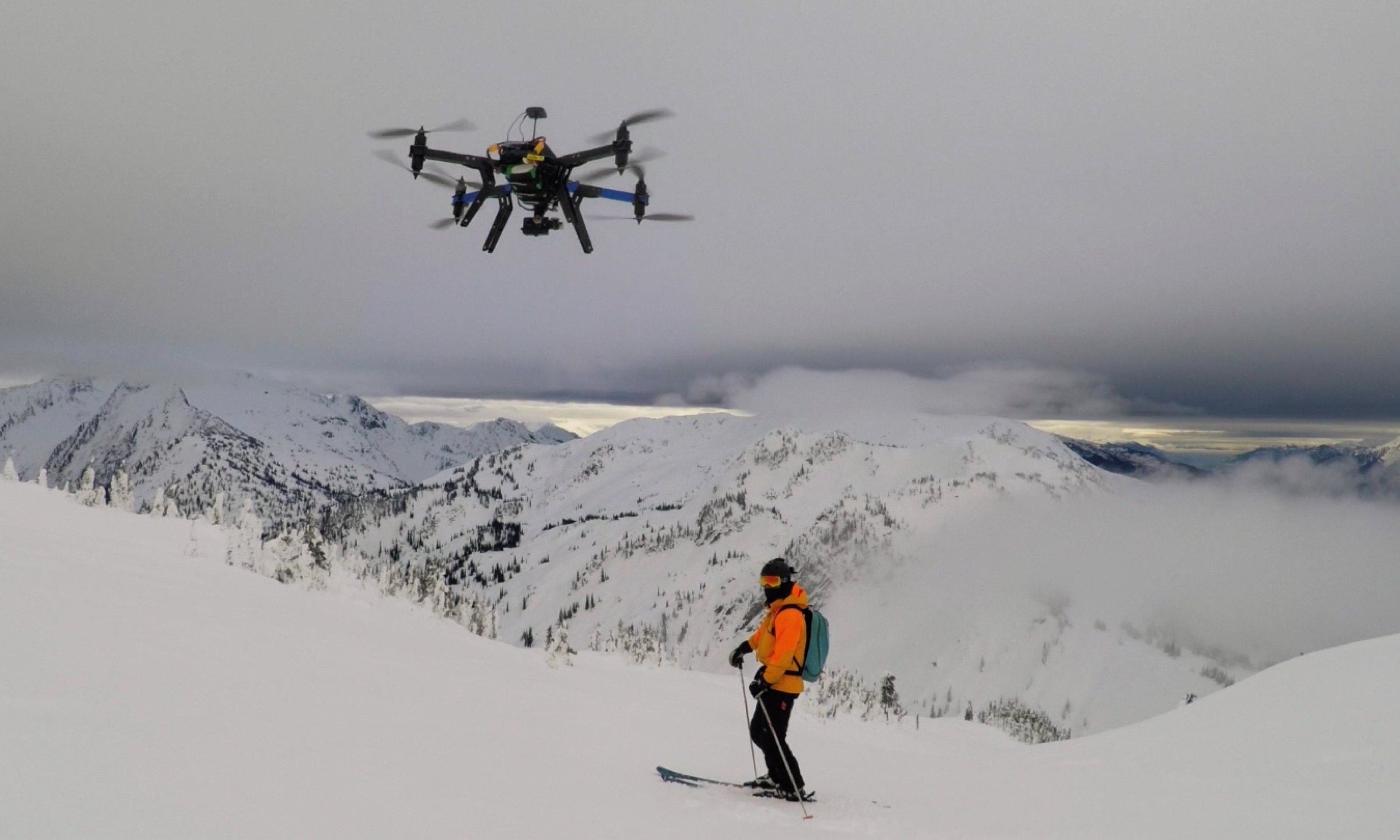In this professional photo taken at the top of a snow-covered mountain at early dawn, a lone skier stands in the foreground, dressed in a bright orange ski jacket, dark pants, and dark gloves, with a dark face covering and hat. He wears vivid orange sunglasses and carries ski poles, while a blue or teal backpack rests on his back. The skier's figure is sharply contrasted by the thick, white snow beneath his feet and the gray, cloud-laden sky above. A typical drone, with multiple propeller arms and a camera attached, hovers overhead, capturing the scene. In the background, a vast mountain range stretches across the horizon, creating the breathtaking impression that the skier is above the clouds, enveloped in a serene, foggy stillness. The subtle hints of sunrise attempt to break through the mist, casting a diffuse light over the majestic landscape, further enhancing the tranquility and beauty of this high-altitude adventure.